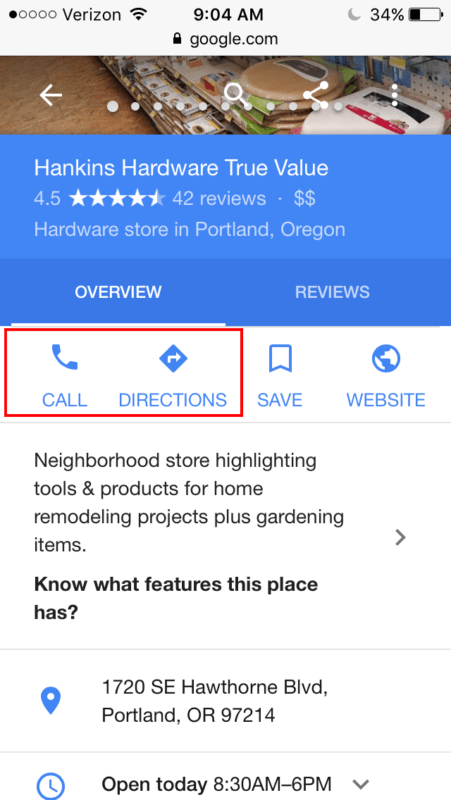The displayed image is a screenshot of an iPhone home screen. In the top-left corner, the network signal shows 1 out of 5 bars, indicating a weak signal, while the network provider is listed as "Version." Adjacent to this, the Wi-Fi signal strength is shown with 3 out of 3 bars, indicating a strong connection. In the top-center, the current time is displayed as 9:04 AM. The top-right corner shows the battery percentage at 34%.

At the top center of the screen, the web address "google.com" is visible. Below this, text in bold advertises "Hankings Hardware True Value," which is rated 4.5 stars based on 42 reviews. It is described as a hardware store located in Portland, Oregon. Several actionable buttons are highlighted, including "Overview," "Reviews," "Call," and "Directions," with "Directions" being highlighted in red. Additional buttons, such as "Save" and "Website," are also displayed.

The store is further described as a neighborhood establishment that offers various tools and products for home remodeling, along with gardening items.